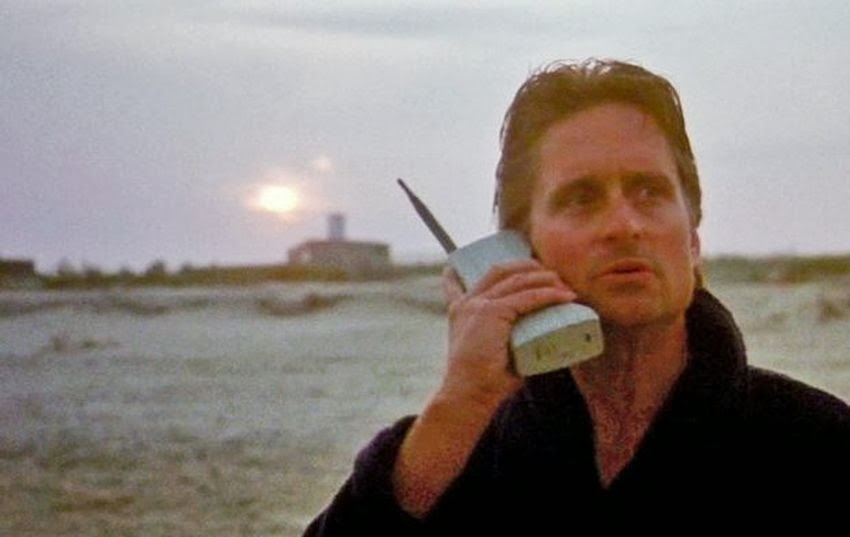In this movie still, actor Michael Douglas occupies the right side of the frame, prominently in the foreground. He is clad in a black bathrobe, his character gripping a large, thick cordless phone—likely from the 90s or early 2000s—with an elongated gray antenna, held to his ear with his right hand. His gaze is directed to the left, looking into the distance as he engages in a conversation. The background, though slightly out of focus and of low resolution, suggests a beach setting with sandy dunes or a desert-like terrain. A hazy horizon indicates either sunrise or sunset, casting a subdued light over the scene. Scattered vegetation, low-lying shrubs or bushes dot the landscape near the horizon, where a building with a smokestack emitting white smoke can be seen. The sky above is clouded and pale, completing the mood of the scene.